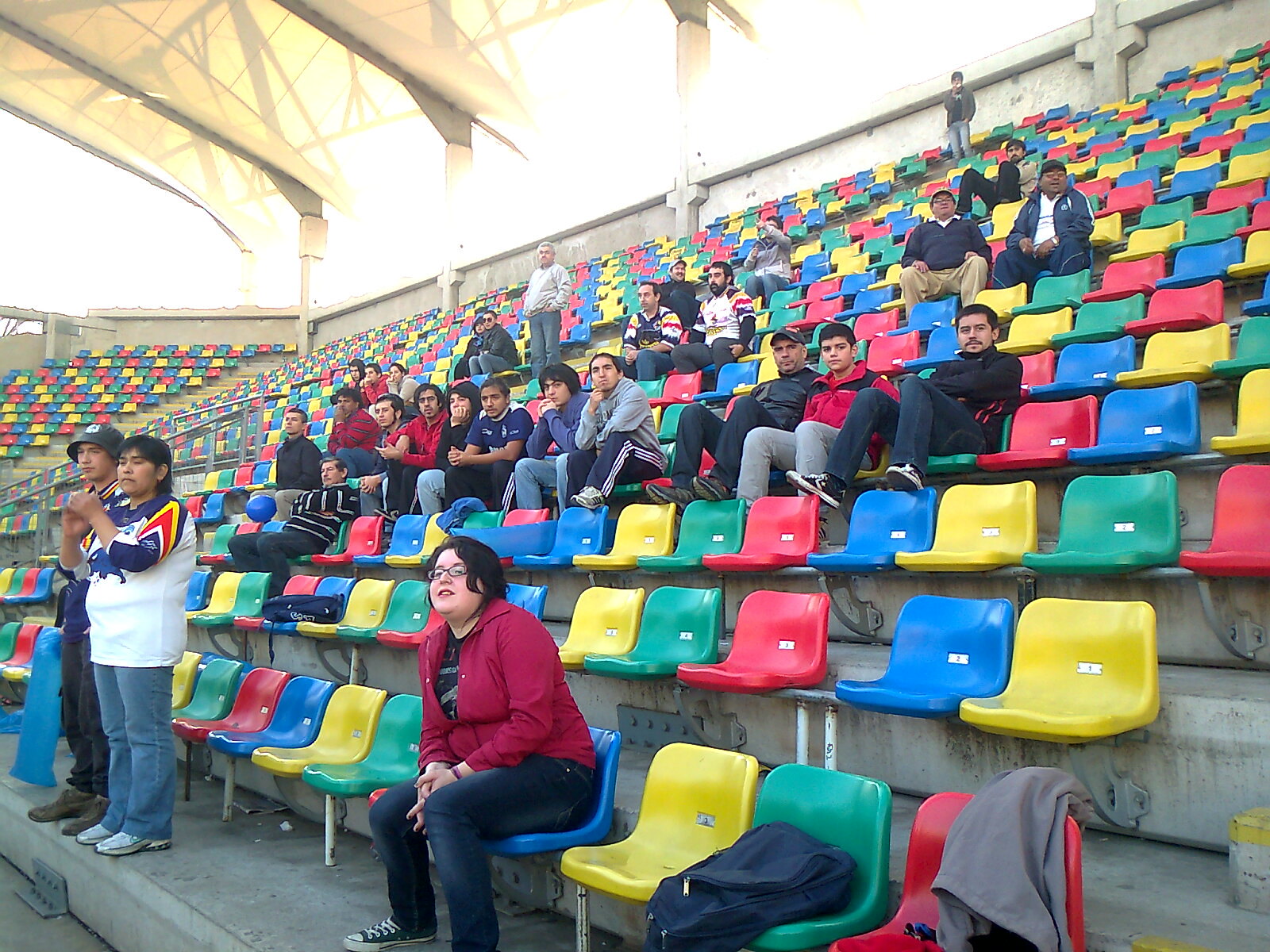The image depicts a vibrant and bustling sports stadium, showcasing a dynamic scene of spectators. The stadium’s seats are laid out in colorful tiers of yellow, blue, red, and green, with concrete steps in a gray hue. The seating arrangement is sporadically populated; some seats are empty, while others are occupied by about 20 to 25 spectators, a mix of males and females. The scene features individuals dressed in various attire, including a maroon jacket worn by a woman in the front row who also has glasses, red and black jackets, jeans, a gray sweatshirt, a multicolored jacket, and white jerseys. The crowd is engaged with the event, with some people cheering and clapping, while others sit or stand in relaxed postures. Above them, an overarching roof provides cover, while the bright daylight illuminates the setting, indicating that the event is taking place outdoors. The background includes a white wall adorned with cross-shaped designs, adding to the architectural detail of the stadium.